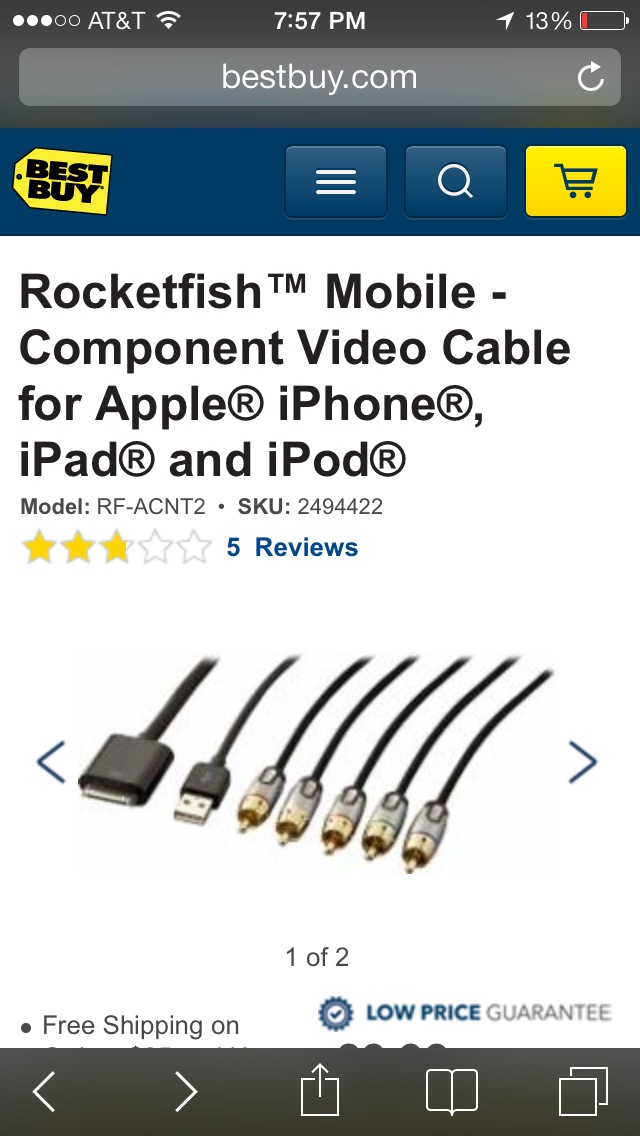The image is a detailed screenshot of the Best Buy website taken on an iPhone, showcasing the Rocketfish mobile component video cables compatible with Apple iPhone, iPad, and iPod (model RF-ACNT2, SKU2494422). The Best Buy logo is prominently located in the top left corner, while a shopping cart icon is placed in the top right. The majority of the screen is occupied by a central display of the various cables for Apple devices. The text highlights information such as "BestBuy.com," "Best Buy," "Rocketfish," and descriptors like "trademark, mobile component video capable for Apple, iPhone, iPad, and iPod," reinforced by keywords like low-price guarantee, free shipping, 5 reviews, and product details.

The screenshot, captured at 7:57 PM with the iPhone showing a low battery at 13%, also indicates a strong Wi-Fi signal but only three bars of internet connectivity. The visual arrangement includes a predominantly white background, accented with dark blue, yellow, black, blue, gray, and traces of red from the low battery indicator, forming a rich, multi-colored composition. The webpage is recognized as being navigated to BestBuy.com, and the overall visual style confirms it as a mobile-optimized screen capture.